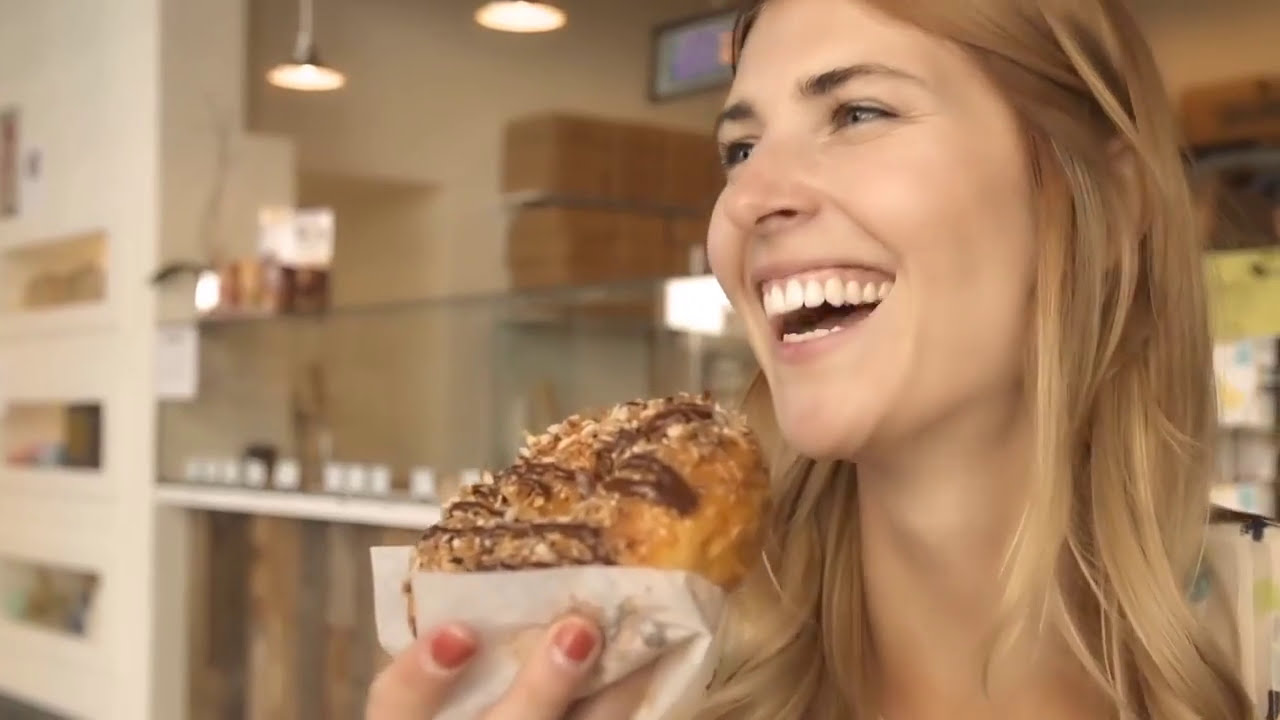The image captures a joyful woman with long, shoulder-length blonde hair and blue eyes, smiling broadly with her mouth open, revealing her top and bottom teeth. She holds a large doughnut adorned with white nuts and a chocolate drizzle glaze in her right hand, her fingers tipped with red nail polish. Positioned to the right-hand side of the frame, she stands in a brightly lit bakery or cafe environment. The background features a slightly blurred but discernible setting, including hanging lamps, a glass barrier atop a counter, and shelves on a white wall to the left. The scene suggests the woman is engaged in a pleasant moment, possibly interacting with someone off-camera.